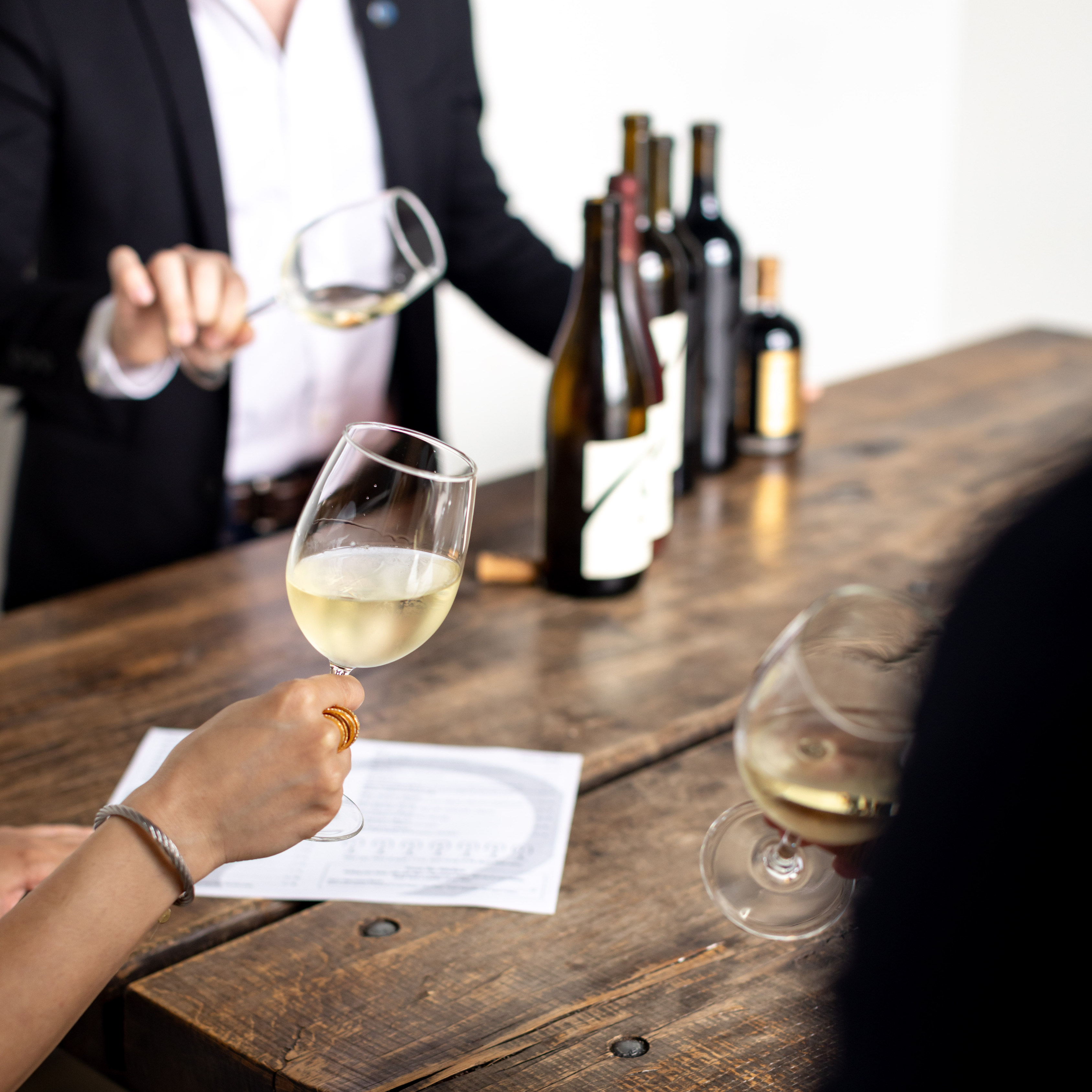The color photograph in portrait orientation captures a detailed scene of a wine-tasting event centered around a rustic wooden table made of two large planks. In the foreground, the bottom right corner features the silhouette of a person's head, seen from behind, holding a tilted glass of white wine towards their face. To the left, a woman’s right hand, adorned with a silver bracelet, also holds a glass of white wine, poised above a white piece of paper that may be for taking notes or scoring the wines.

The tabletop is populated with about five mostly out-of-focus wine bottles of different colors and brands, lined up side by side, accompanied by a shorter bottle. In the background, slightly to the upper left of the scene, a man dressed in a black blazer and white button-up shirt stands. His torso is visible from the shoulders to the waist. He is rotating a glass of white wine in his fingers, with the glass nearly horizontal, as if about to pour it out.

The setting is brightly lit with natural light, enhancing the clarity of the image and the intricate details of the scene, contributing to a realistic and representational style.